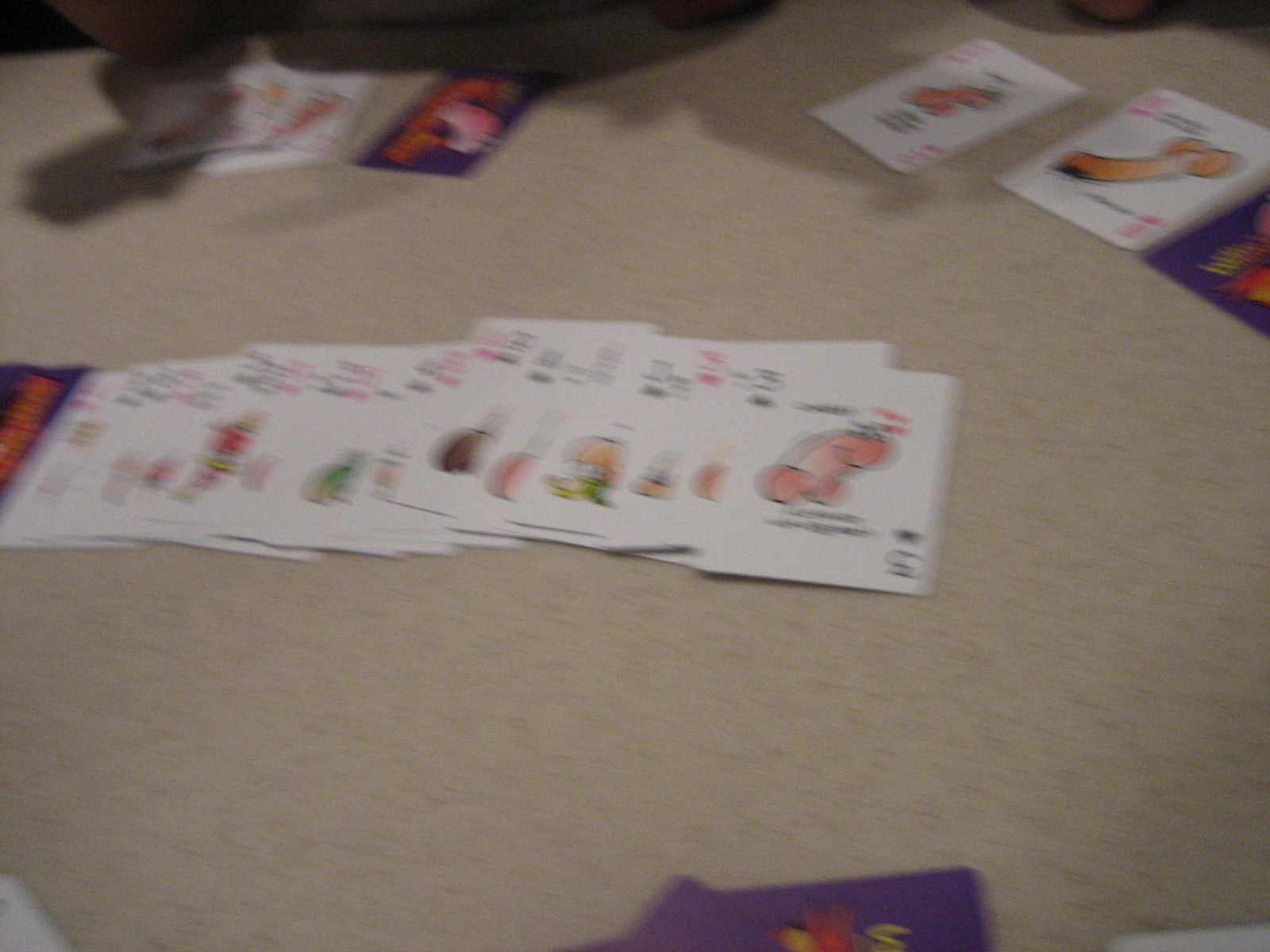The photograph depicts a heavily blurred and poor-quality indoor scene centered around a collection of assorted cards scattered across a light tan-colored floor. In the upper left corner, the vague shadow of a person can be discerned on the floor, hinting at human presence. Several white cards, approximately the size of standard playing cards, occupy this section, their images indistinct due to the blurriness.

To the right of these white cards, a purple card appears, similarly blurred and unreadable. The upper right-hand corner reveals two more white cards alongside the partial view of another purple card, though their details remain elusive.

The central focus of the image features a horizontal line of playing cards fanned out, displaying various images and undecipherable numbers in their corners. The final card in this sequence, positioned to the far right, might show the number five, though clarity remains compromised.

In the lower section of the photograph, particularly towards the middle, a few more purple cards are visible, partially emerging from the bottom edge of the frame. The overall scene, though rich in potential details, is greatly obscured by the remarkable level of blur, making precise identification challenging.